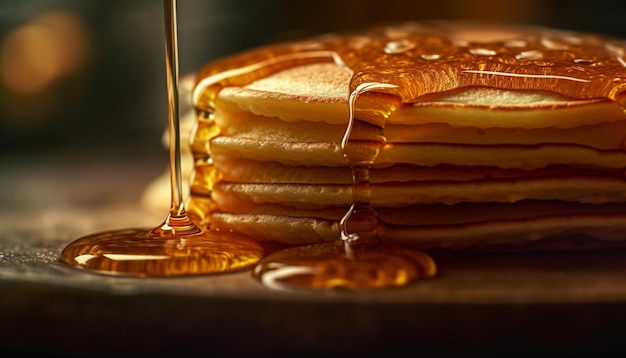This is an up-close promotional photograph of a stack of four medium-size, golden brown pancakes set on a dark brown wooden table. The pancakes display a gradient of colors with a perfectly brown center, a pale ring, and a crispy, dark brown edge. A generous amount of amber-colored, light brown syrup has been poured over the stack, forming a blob on the top pancake and cascading down in two visible streams. The syrup pools onto the plate and table surface, creating a visually appealing scene. The background of the photograph is blurred, keeping the focus on the deliciously inviting pancakes and syrup.